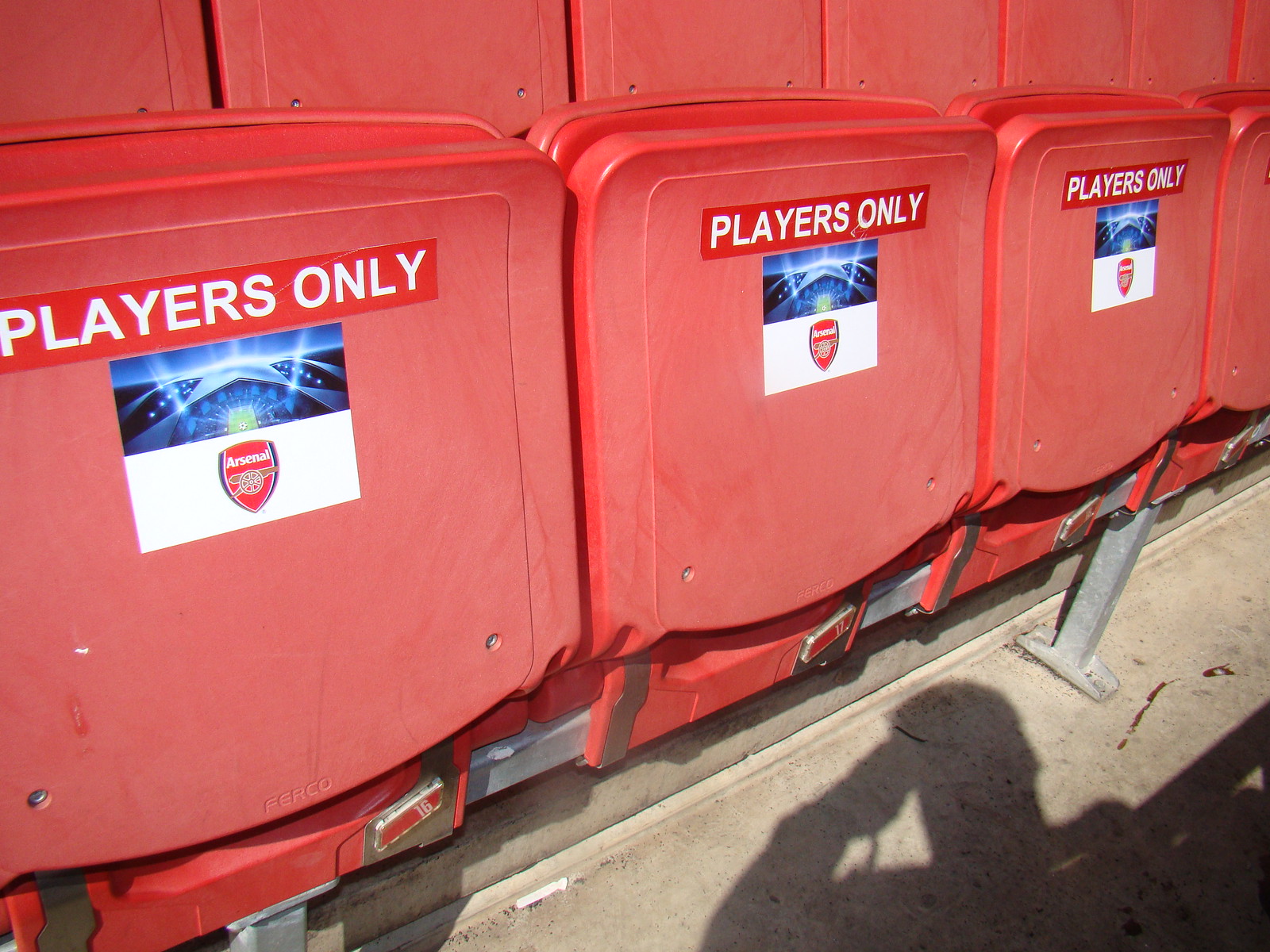The image depicts two rows of red plastic bleacher seats in a sports stadium, likely designed for players, as indicated by the "PLAYERS ONLY" labels with white text on a red background affixed across the seats. The seats are weathered, suggesting they are sun-worn and have been exposed to the elements. They are the type that automatically flip up when not in use. At the bottom of the frame, concrete flooring and metal framework are visible, supporting the bleachers. Centrally located among the seats is a decorative image featuring a futuristic soccer stadium with a white box underneath displaying the badge logo of the sports team Arsenal, which includes a small illustration of a brown cannon.